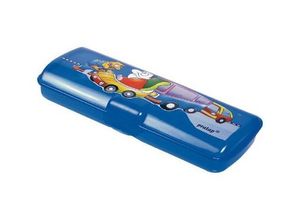The image showcases a simple, blue plastic pencil case placed against a white background, tilted slightly to the side with the opening facing left at an angle, though it remains closed. The design on the lid consists of a cartoonish decal. Dominating the illustration is a character with a pronounced nose driving what appears to be a small bumper car. This car has a green backrest and is followed closely by a blue bus with a purple top, as well as a red and yellow vehicle that could be the back of a station wagon or trailer. Additionally, there is a mechanic-like figure standing to the left, observing the driver. Above this scene, the brand name "PRATAP" (or possibly "PruTap") is printed with a copyright or trademark symbol. The design appears to be a sticker applied to the pencil case, which measures roughly eight inches in length, three inches in depth, and one inch in height. There is a slight glare on the plastic surface, enhancing its shiny blue color.